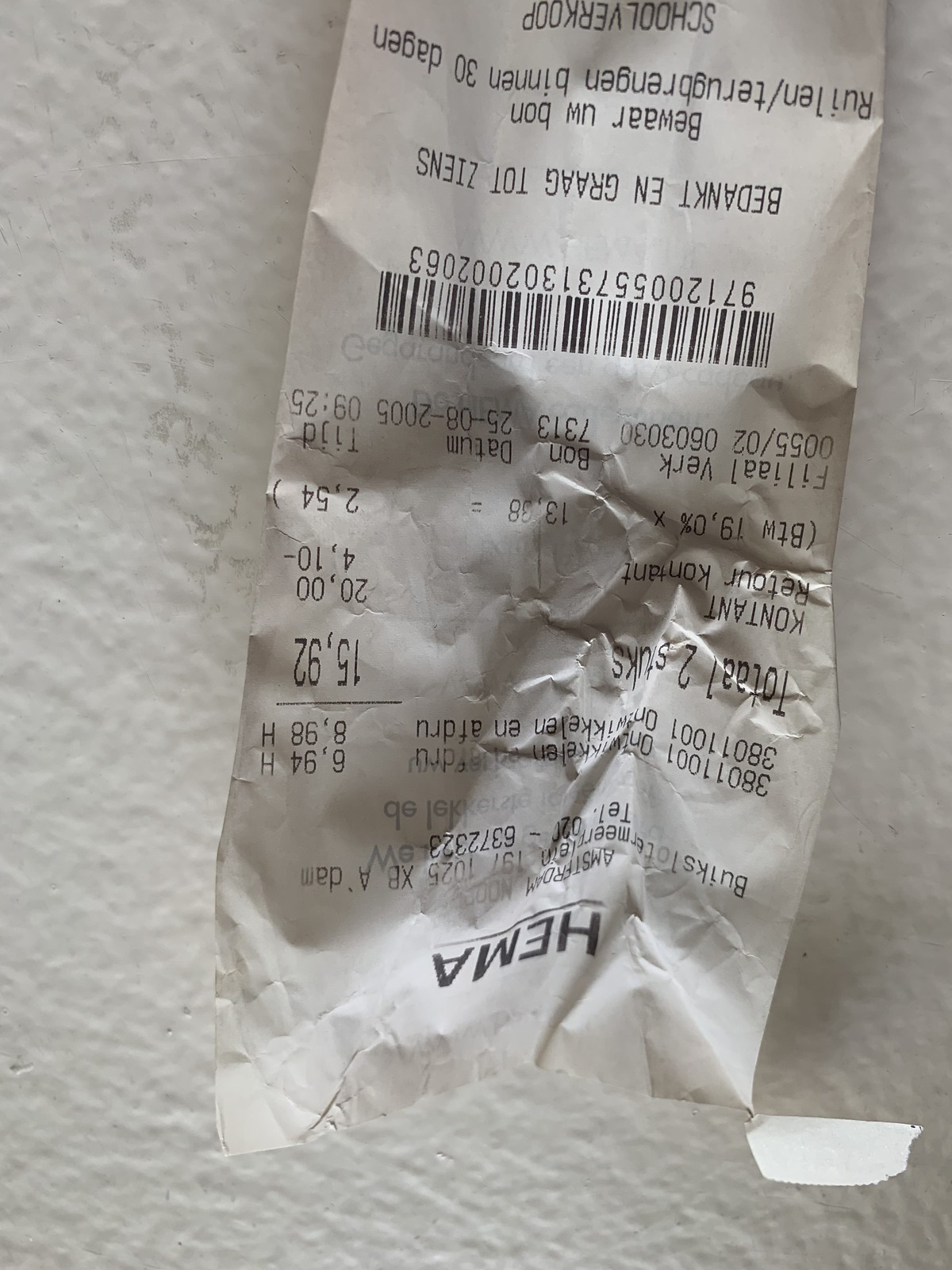A wrinkled receipt lies centered on a white, nubby-textured surface. Printed in black font, the business name "H E M a" prominently appears at the top, accompanied by several numbers and a phone number. The receipt lists two purchased items, one costing $6.94 and the other $8.98, bringing the total to $15.92. Towards the bottom, a barcode and a string of numbers are displayed. The text on the receipt is written in a foreign language. The sole focus of the image is the receipt on the textured backdrop, with no additional objects in sight.